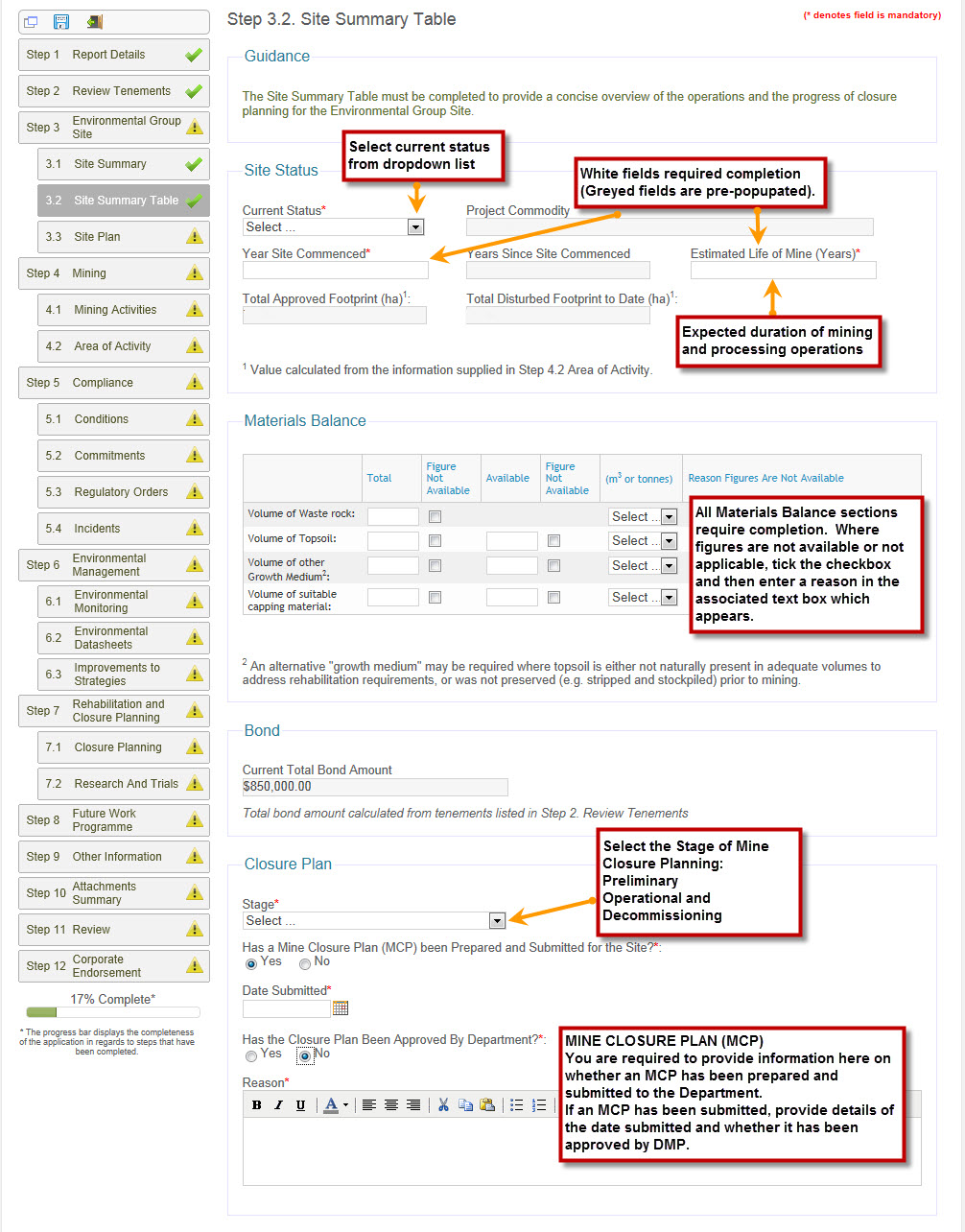This image is a detailed view of a "Site Summary Table" as part of step 3.2 of a larger documentation or report. Although the company name is not present, the table is organized into several sections with distinct color codes and interactive elements. 

- At the top, there is a blue "Guidance" section, followed by an equally blue "Site Status" section. 
- Below these sections, there are blue-labeled areas for "Materials Balance," "Bond," and "Closure Plan." 
- Each section contains detailed text encapsulated within red boxes with black lettering. Additionally, interactive drop-down menus are integrated within these sections, creating a cohesive flow from top to bottom.

On the left side of the image, there is a gray-shaded sidebar labeled with fields such as "Report," "Report Fields," and "Review Testaments." This sidebar is densely populated with information within gray boxes, with one box being a darker shade of gray. 

Towards the bottom of the page, a progress bar is visible, displaying "17% compatible" with a green bar extending to the right. 

Lastly, at the very bottom, there is a section labeled "Reason," which includes a text entry area for adding supplementary information.